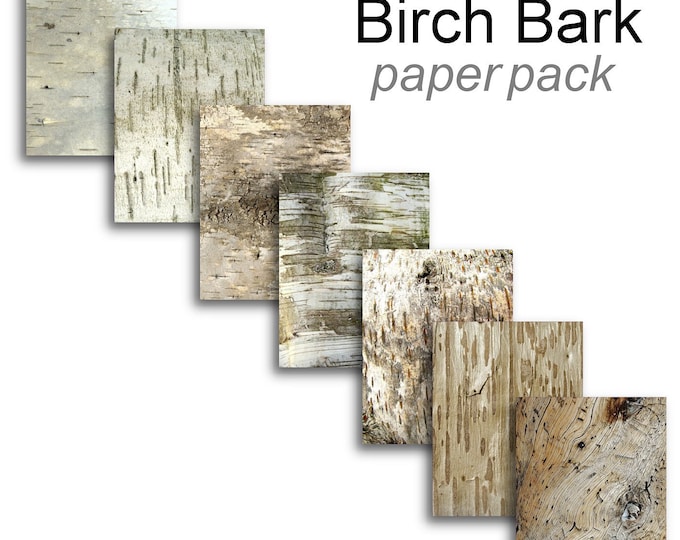The image features a minimalist design with a plain white background. In the top right corner, bold black text reads "Birch Bark," with the B's capitalized. Just below, in italic gray lowercase font, it reads "paper pack." Arranged diagonally from the top left to the bottom right are seven rectangular pieces of birch bark paper. The top-left piece is light gray with scattered black lines. Each subsequent piece shares a similar light gray hue with vertical lines, transitioning through varying shades of gray and brown. The progression includes off-white, tan, khaki, and hints of olive green, culminating in a much darker brown piece that is cut off at the bottom. The pieces are arranged in a staggered, staircase-like layout, overlapping slightly to display their unique, wood-like patterns and textures. This image is likely used for marketing, perhaps as a decorative paper pack for craft projects or cards.